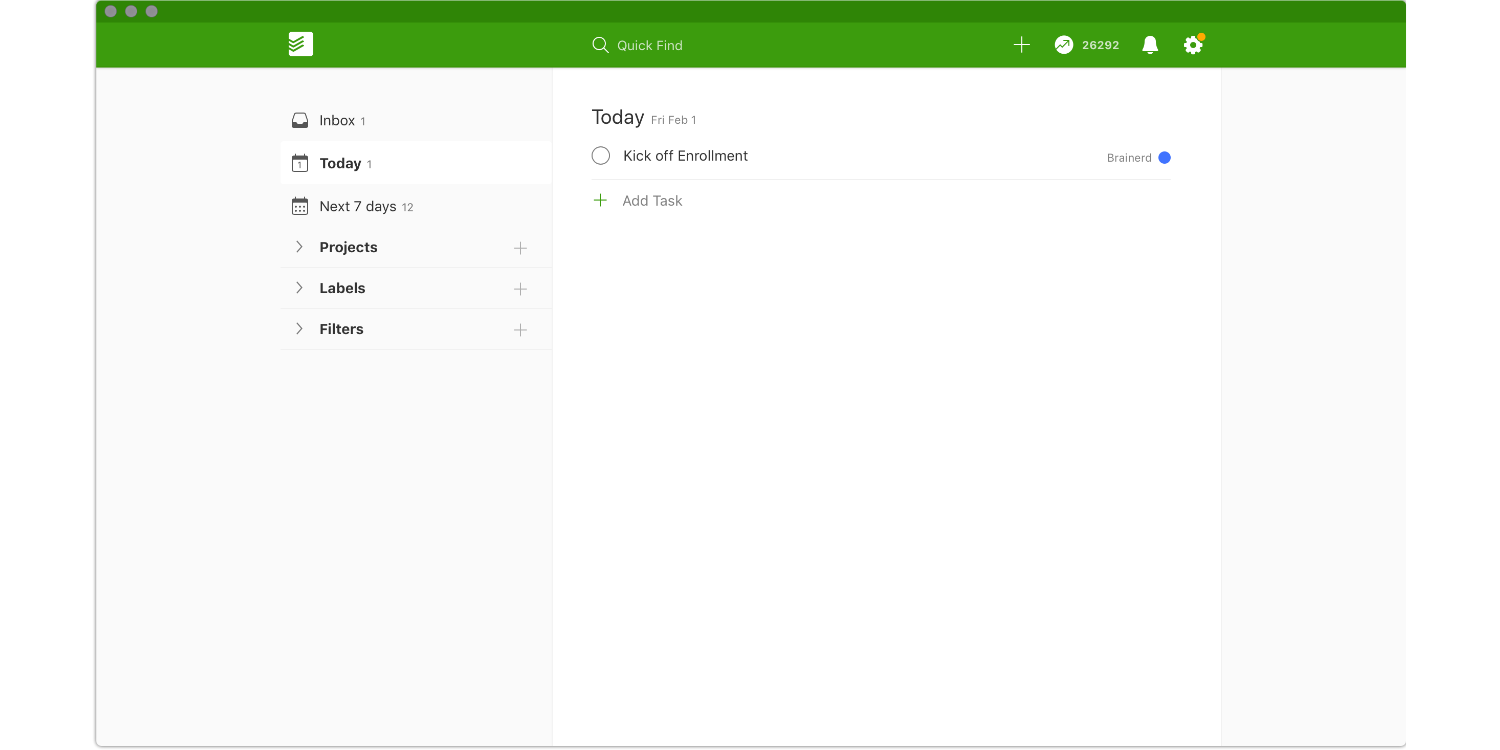The image appears to be a screenshot of a web application interface, captured from a computer screen. The top of the page features a header with a dark green upper section transitioning to a brighter green lower section. On the upper left side of this header, there are three horizontally-aligned gray dots. Below the dark green section, a light green bar contains a series of icons: a white square with three ticks on the left, a magnifying glass icon labeled "Quick Find," a plus symbol, a small graph-like icon with an arrow pointing upwards to the right and the number 26292, a bell icon, and a gear icon with a small orange dot at its upper right.

Beneath the header, a sidebar on the left has vertical tabs on a light gray background, which include: "Inbox 1," "Today 1," "Next 7 Days 12," "Projects," "Labels," and "Filters." Each of these tabs is accompanied by a gray plus icon to the right and a gray arrow icon to the left, pointing rightwards.

The main content area of the page, set against a white background, displays minimal information. It reads, "Today, Friday, February 1st," followed by a black-outlined circle with a white center labeled "Kickoff Enrollment." To the right of this text, the term "Brain Nerd" is displayed alongside a blue dot. Below this, a horizontal light gray line separates the text from an area featuring a green plus icon and the label "Add Task" in light gray.

The page does not provide explicit details regarding its application type, but given the presence of terms like "Inbox," "Today," and "Add Task," it might be a productivity or event management tool, rather than a traditional calendar app. The exact purpose of the application remains ambiguous from the screenshot alone.